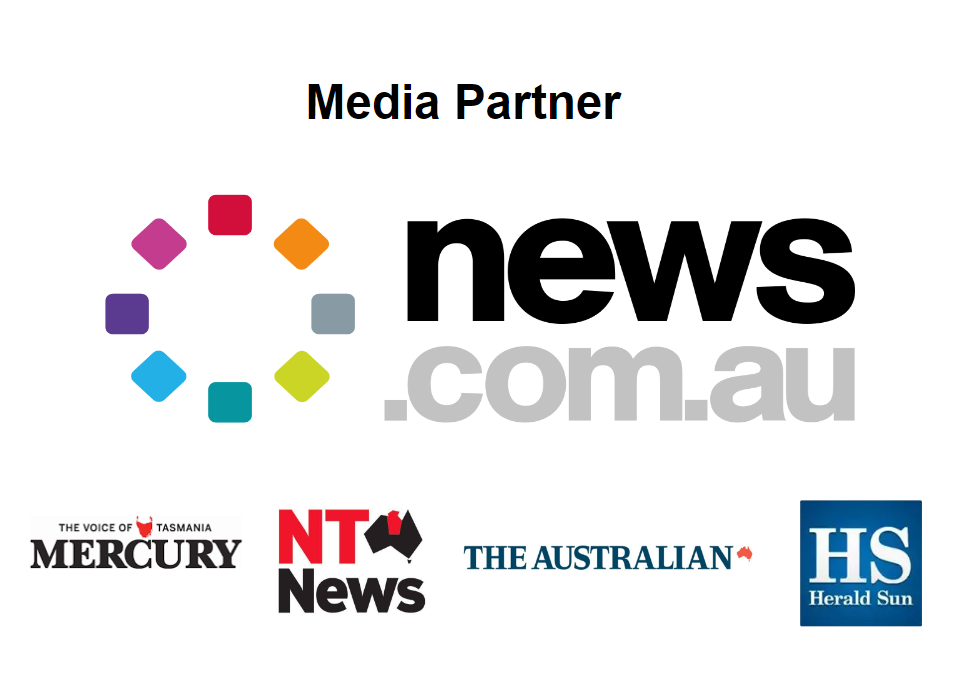The image showcases a collection of media partner logos and icons against a white background. At the top, in bold black text, the words "Media Partner" are prominently displayed. The central section features the logo for news.com.au, consisting of eight rounded squares in different colors arranged in a circular pattern, with "news" in black and ".com.au" in gray, all in lowercase.

Below the news.com.au logo, there are additional logos representing various Australian news outlets, arranged from left to right:

1. **The Voice of Tasmania**: The logo includes the phrase "The Voice of Tasmania" in smaller capital letters above the word "Mercury" in large, bold, black capital letters. To the left of "Tasmania," there is a red silhouette of Tasmania Island.
   
2. **NT News**: The "NT" part of the logo is in red capital letters, while "News" is in black capital letters. There is also a graphic of Australia with the Northern Territory outlined in red.

3. **The Australian**: The logo is set in all capital letters with a red silhouette of Australia to the right of the text.

4. **Herald Sun**: This logo features a blue square with white text. The letters "HS" are prominently displayed in large, capitalized font in the center, with the words "Herald Sun" underneath.

Each of these logos collectively represents a diverse array of Australian news outlets, highlighting their partnerships and media connections.